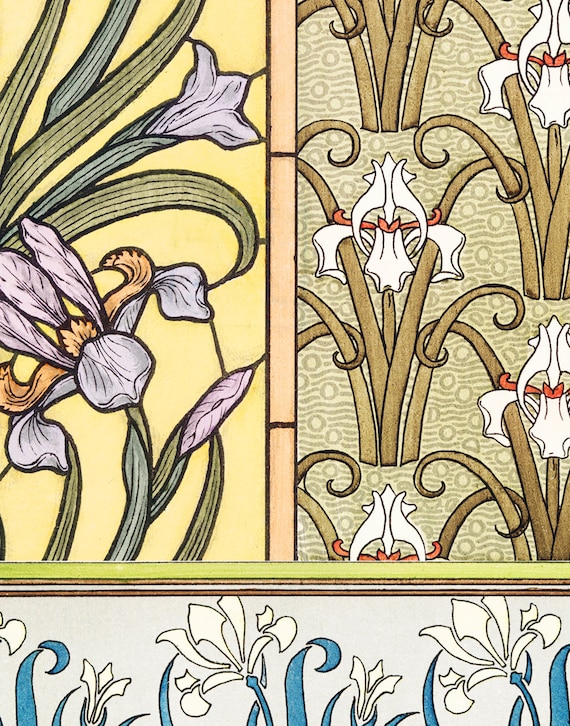This image showcases an intricate, Art Nouveau-style color illustration divided into three distinct sections. The overall illustration is set in portrait orientation. The upper two-thirds of the image are split into two vertical panels, while the bottom third is a horizontal band stretching from left to right.

The upper left panel features a portrait-oriented design with a light yellow, almost cream background. Here, the foreground is dominated by irises, their petals rendered in soft lavender hues. The stems and leaves are depicted in a mix of olive greens and muted blues, intertwined with an additional central vertical band of segmented peach color.

To the right, the upper right panel also follows a portrait orientation and is more dynamic with circles and wavy lines reminiscent of water. This segment hosts white irises with eye-catching red centers or center leaves. The stems are primarily brown, adding an earthier tone to the composition.

The bottom horizontal band contrasts yet complements the top sections with its bluish background. This section is adorned with blue leaves and white flower petals, stenciled delicately against the backdrop. The interplay of soft colors and rhythmic patterns across all sections unifies the piece, drawing from the shared motif of irises and reflecting the detailed craftsmanship typical of Tiffany glass designs.